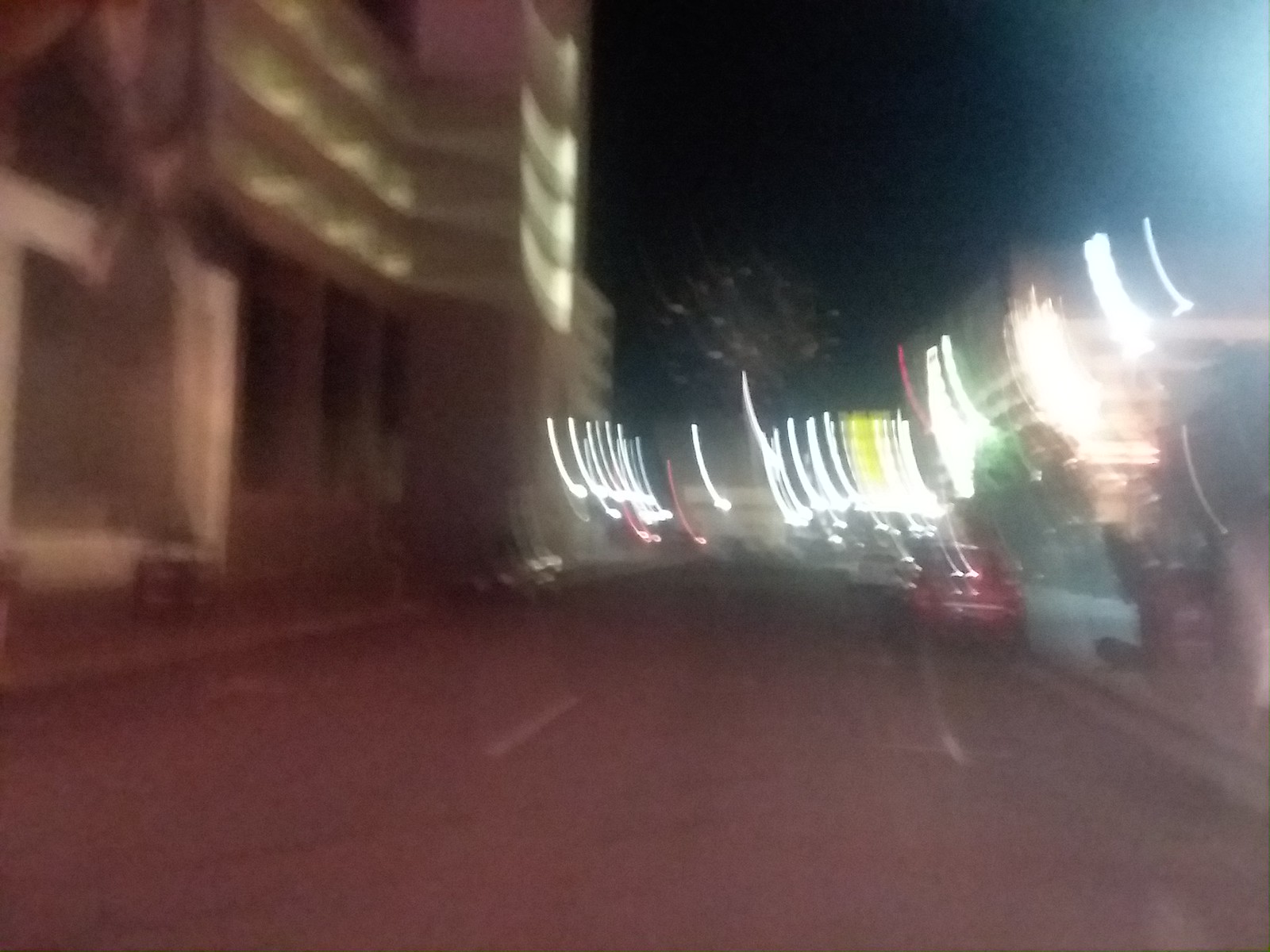A heavily blurred image taken in a town centre, possibly either accidentally or in jest, mimicking the perspective of someone with astigmatism. The photo predominantly features streaks of lights going up and down, obscuring clear visuals. In the foreground, a red car is parked in front of a building. To the left, another building appears closed and unlit, with a banner hanging across its top. The centre background may contain a tree, although it’s hard to discern due to the blurriness. Road markings and parking bays are also visible, adding to the urban setting context.